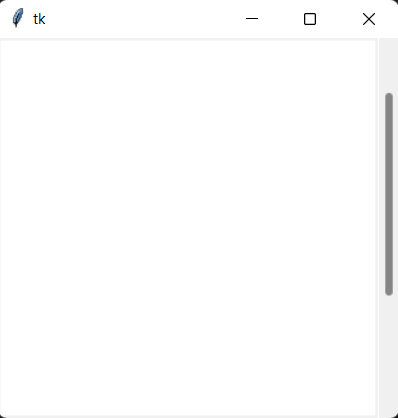Screenshot Description: 

The image is a small, ambiguous screenshot that lacks significant contextual information, making it unclear whether it is from a webpage or a cell phone display. Dominating the top left corner is a small gray triangle, next to which a black feather-like icon is situated. Adjacent to this, the lowercase alphabetical characters 't' and 'k' are visible.

The far right of the image features standard window control icons: a black minimize button, a black square representing the maximize/restore function, and a black 'X' for closing the window. A black triangular section occupies the upper-right corner of the screenshot.

A light gray horizontal line spans the width of the image below these elements. On the right-hand side, running vertically from the bottom to the top, is a light gray area housing a darker elongated oval shape resembling a scrollbar. At the bottom right corner, another darker gray triangle is present.

Additionally, a horizontal gray line runs along the bottom edge of the image. The left lower corner contains a very small dark triangular shape nestled into the edge. The central part of the image is largely blank, contributing to the overall paucity of detailed content.